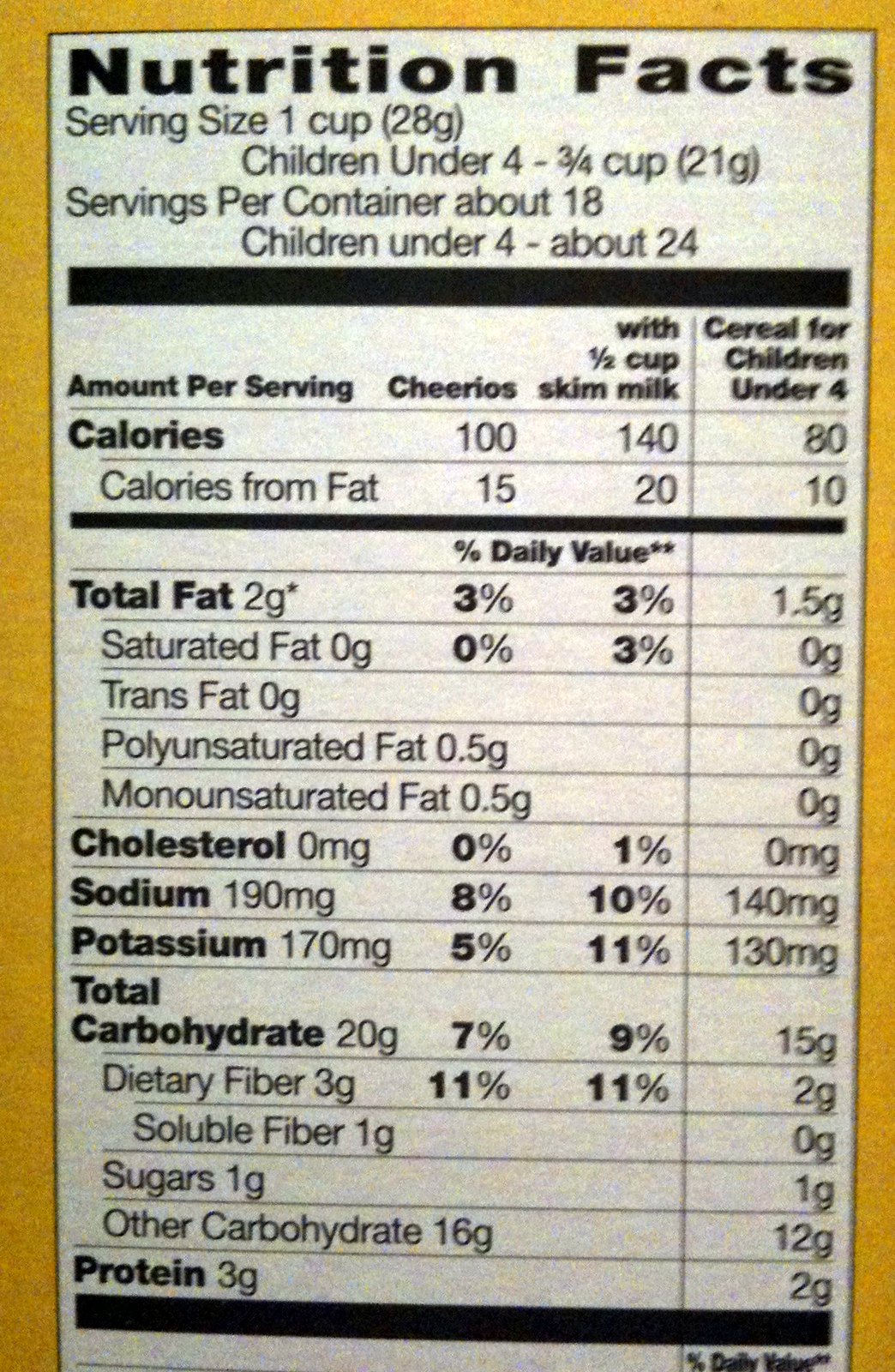The image features a detailed nutrition label, presented in black and white, set against a vibrant yellow background. The label, presumably printed on the side of a Cheerios cereal box, provides comprehensive nutritional information per serving. At the top, it prominently displays "Nutrition Facts," followed by serving sizes: one cup (28 grams) for adults, and three-fourths of a cup (21 grams) for children under four years old. The container offers 18 adult servings or approximately 24 child servings. The label further details caloric content: 100 calories from just the cereal, 140 calories when combined with one-half cup of skim milk, and 80 calories per child serving. Caloric contributions from fat are also listed: 15 calories from fat for the cereal alone, 20 when paired with skim milk, and 10 for child servings. Additionally, the label breaks down various fat contents including saturated fat, trans fat, polyunsaturated fat, and monounsaturated fat, alongside cholesterol, sodium, potassium, total carbohydrates, dietary fiber, sugars, and protein values.